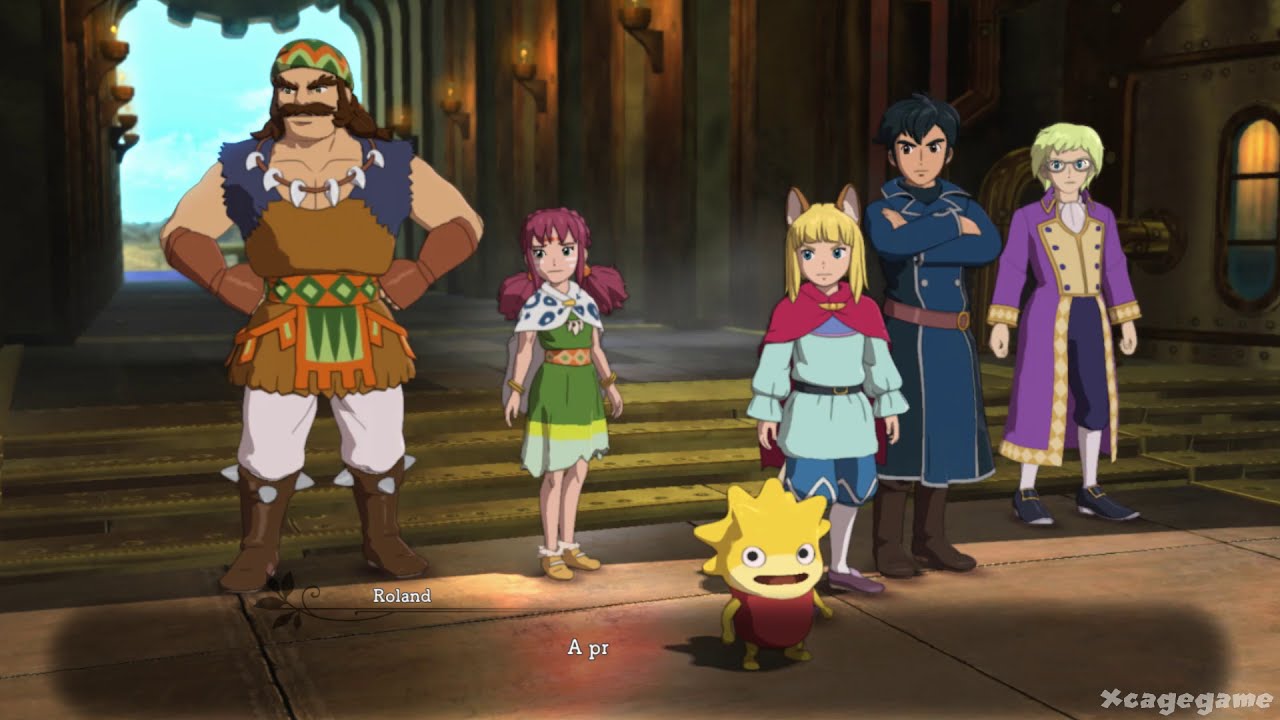This horizontal-rectangular cartoon image, set inside what appears to be a castle interior, features six distinct characters. On the left stands a large man with a big, brown mustache, long hair, and wearing medieval-themed attire, including a leather singlet, brown gloves, and spiked boots. He appears stern with his hands on his hips and a necklace that looks like it's made of teeth. Next to him is a small girl with purple hair in two pigtails, dressed in a little green dress with a white shawl and beige shoes. Prominently in the foreground is a small, spiky yellow-haired boy with a red shirt, spiky hair, a round head with protruding spikes, far-apart eyes, yellow limbs, and a mouth agape, giving him a turtle-like appearance. To the right stands a girl with blonde hair and cat ears, dressed in a blue outfit with white tights and flats. Next to her is a man with dark hair, arms crossed, wearing a long blue coat with a brown belt and dark brown boots. On the far right is a slender figure with glasses, blonde hair, and dressed in a long purple coat or jacket, layered over purple and white tights, wearing leather footwear. The background shows steps leading up to an open door, with the words “Cage Game” and an “X” symbol visible at the bottom right of the image. The two characters on the left side of the image appear quite unhappy.